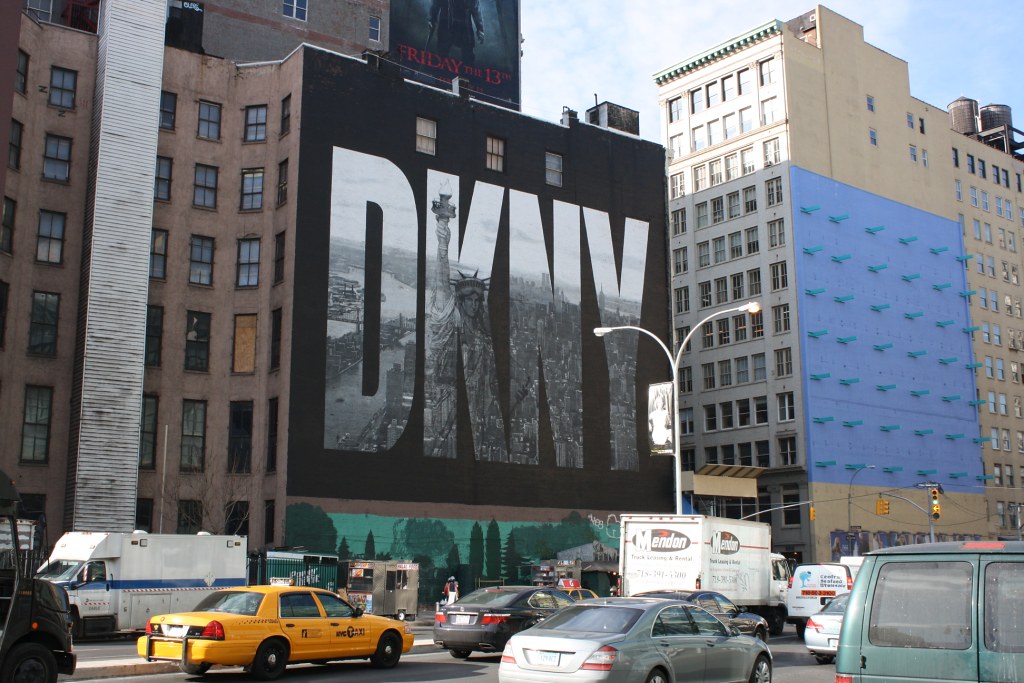This vibrant daytime photo captures a bustling cityscape from the perspective of someone standing on one side of a busy street. Multiple lanes of traffic stretch out before us, filled with vehicles traveling away. A notable formation of vehicles includes a van, a yellow taxi, a white truck, a white van, and several other cars. Across the street, an ambulance is parked and facing the opposite direction, adjacent to a visible food truck. Looming large on the other side, a building prominently displays a DKNY advertisement on a black background; the ad itself is a creative depiction featuring a New York cityscape with the iconic Statue of Liberty. Another towering multi-storied building, characterized by its blue and brown facade, completes the urban tableau.